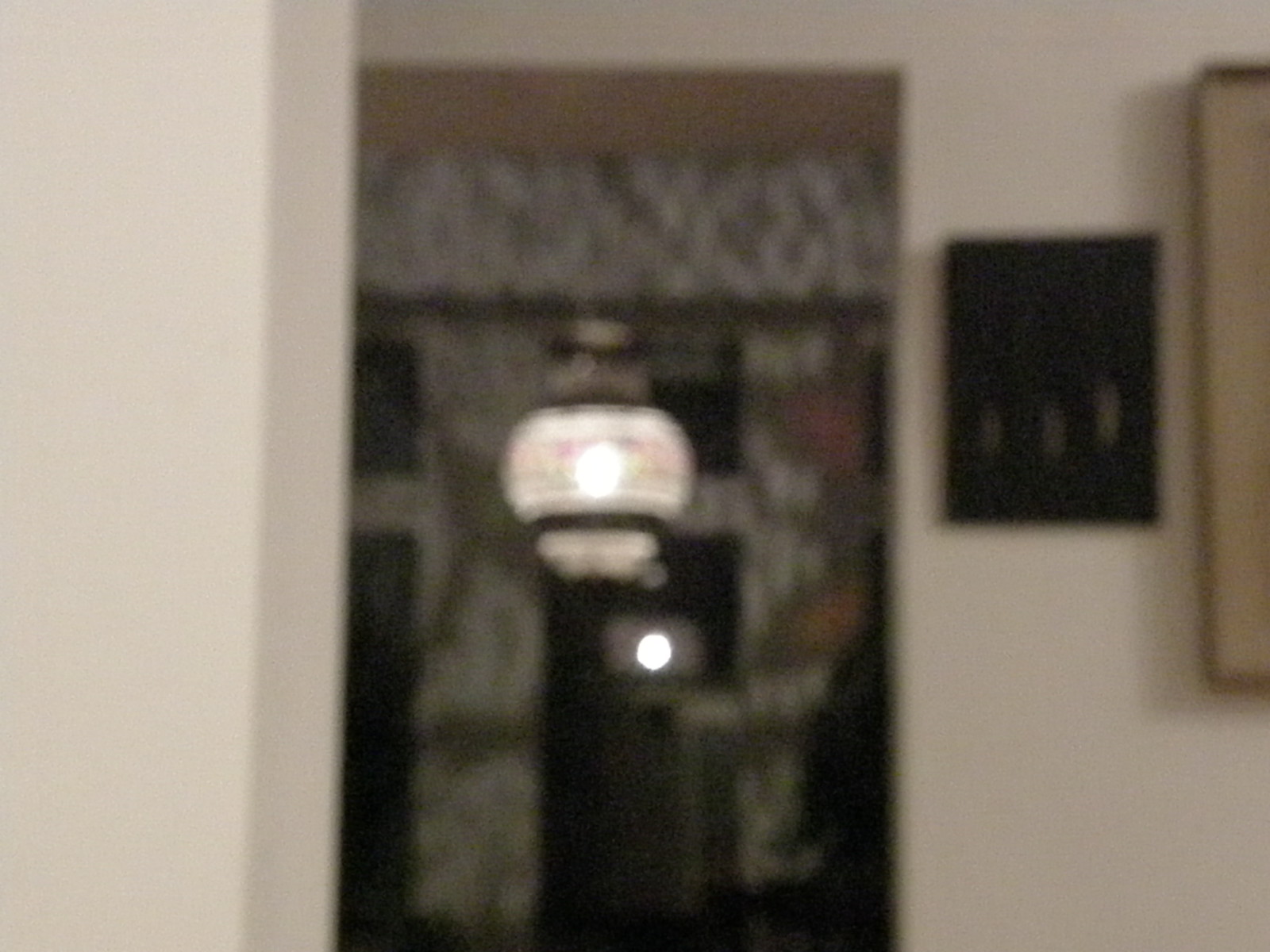This image, captured indoors, depicts a view from one room into another within a house. Despite its blurriness and light glare, key elements can be discerned. The left and right walls of the initial room are white, with the left side completely bare and the right side featuring a black, rectangular picture frame. Another visible frame appears beige, though only partially seen. Dominating the middle section is a walkway leading into a second room. This adjacent room features beige walls and windows adorned with curtains—likely gray and white—though their patterns are indistinguishable. From the ceiling, a round, bulbous pendant light with white and red hues hangs prominently. The scene captures elements like a bulbous ceiling light and the transition between two rooms, emphasizing the interior decor through its white and beige color palette.